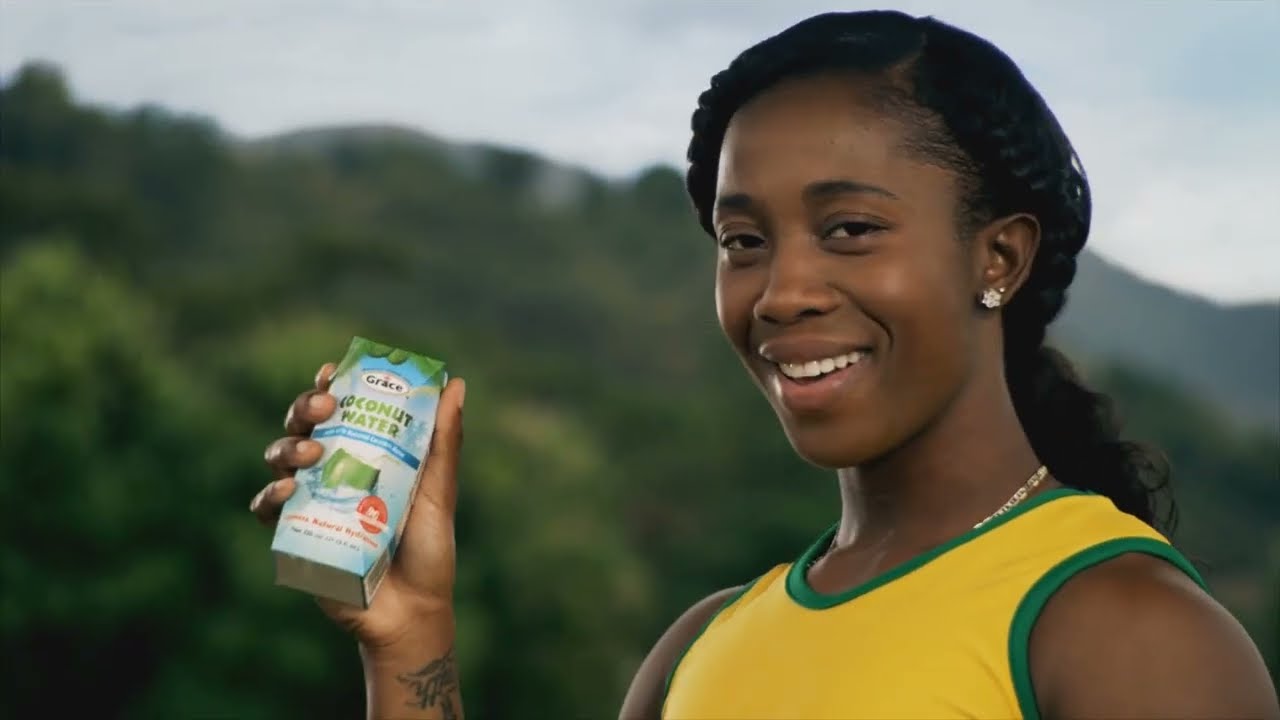A detailed photo shows a young black man with short, close-cropped hair and a dark button earring in his right ear, drinking from a clear plastic bottle labeled "Apple Cider." The label on the bottle is predominantly yellow and green, and the drink inside has a yellowish-orange hue, resembling apple cider or a similar fruity beverage. He holds the bottle in his left hand and is taking a sip, with the bottle raised to his lips. He is dressed in a black-and-white plaid shirt with an open collar and appears to be sitting on a couch in a living room. The couch features a mix of light orange, yellow, and possibly some red colors. The room has a green wall and a bright light situated in the upper right-hand corner, casting a blur over the background. The main focus of the image is the man enjoying his drink.